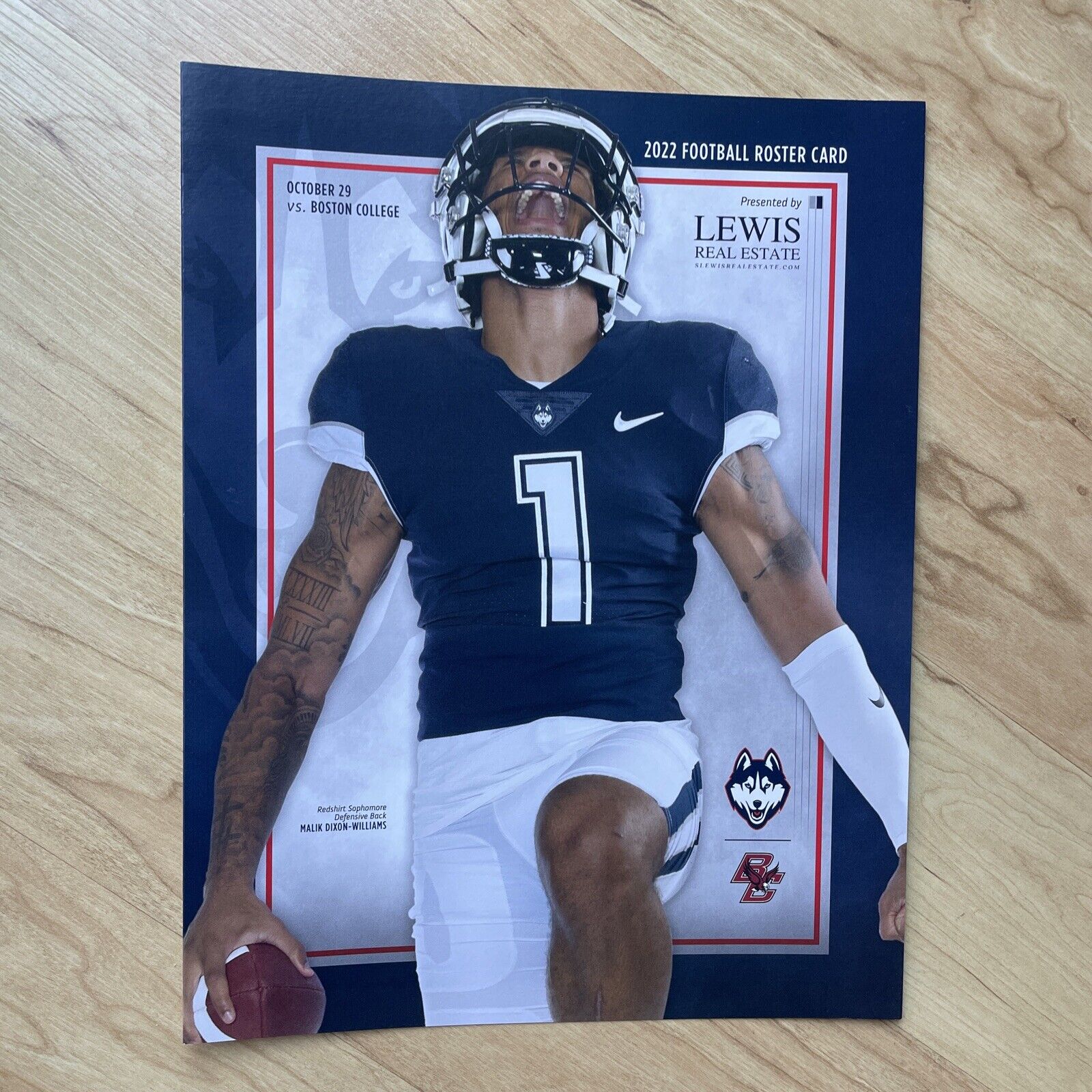This detailed poster, likely a 2022 Football Roster Card, prominently features UConn's redshirt sophomore defensive back, Malik Dixon-Williams, wearing a dark blue Nike jersey marked with the number one. The image captures Malik energetically with his mouth wide open in a spirited yell, his head tilted back while he holds a football in one hand. His highly tattooed arm is also noticeable. The player dons a white helmet, and one knee is raised.

The upper right corner of the poster showcases an advertisement for Lewis Real Estate and states "2022 Football Roster Card." The lower right features the Boston College logo alongside a wolf, presumably the team's mascot. The caption announces a game on October 29th versus Boston College. This visually striking card, with a blue border and a background showing a brown wood-grain surface, serves both as a collectible and a game-day promotional material.